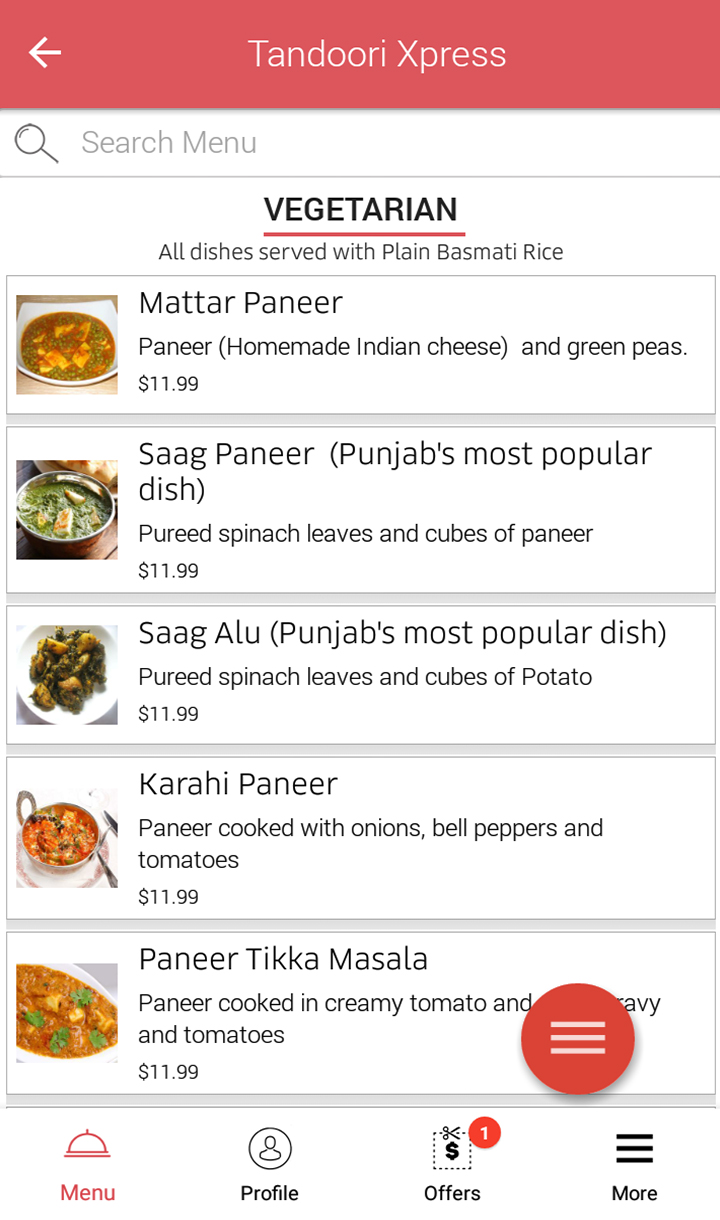The image depicts a phone screen displaying the menu of a restaurant named Tandoori Express. The menu is surrounded by a red border at the top, featuring a small arrow pointing to the left and the restaurant's name prominently displayed in the center. Directly below this, there is a magnifying glass icon accompanied by the text "Search Menu." Following this is the heading "VEGETARIAN" in all caps, underlined in red, and beneath this, the text states "All dishes served with plain basmati rice."

On the left side of the screen, there are images of various dishes accompanied by descriptions and prices. The first image is of a bowl containing Matar Paneer, described as homemade Indian cheese (paneer) and green peas, priced at $11.99. Below this, there is a photo of another bowl labeled Saag Paneer, noted as Punjab's most popular dish, consisting of pureed spinach leaves with cubes of paneer, also priced at $11.99. 

The third option is a plate of Saag Aloo, another of Punjab's popular dishes, featuring pureed spinach leaves with cubes of potato, priced at $11.99. Next, a photograph shows a bowl with reddish and brownish food, identified as Karahi Paneer, which consists of paneer cooked with onions, bell peppers, and tomatoes, priced at $11.99.

Further down, there is an image of a plate with both brown and green elements labeled Paneer Tikka Masala, described as paneer cooked in creamy tomato sauce. Unfortunately, a red dot obscures part of this text, making it partly unreadable. This dish is priced at $11.99.

At the bottom of the page, there are icons for Menu, Profile, Offers, and More, providing navigation options for the user.